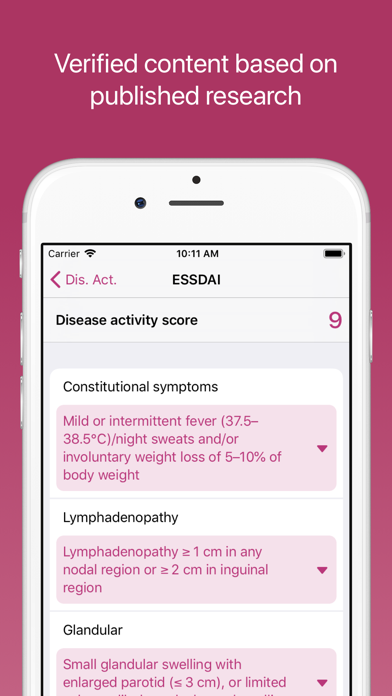A promotional graphic features a hot pink box approximately the size of a phone screen, with bold white text stating "Verified Content Based on Published Research." Within the pink box, an iPhone appears partially visible, with its lower portion cut off near the thumbprint sensor. The iPhone's screen displays several icons and text details: it shows full Wi-Fi signal, the time 10:11 AM, and a fully charged battery icon. The interface indicates the user is in an app with a back arrow labeled "D.I.S. A.C.T." and is currently viewing the "E.S.S.D.A.Y." section. The screen reads, "Disease Activity Score is 9," followed by detailed medical symptoms including, "Constitutional symptoms: mild or intermittent fever, night sweats, and/or involuntary weight loss (5-10% of body weight)." Further details include, "Lymphadenopathy: less than 1 cm in any nodal region or ≤2 cm in the inguinal region," and "Glandular: small glandular swelling with enlarged parotid, less than 3 cm."